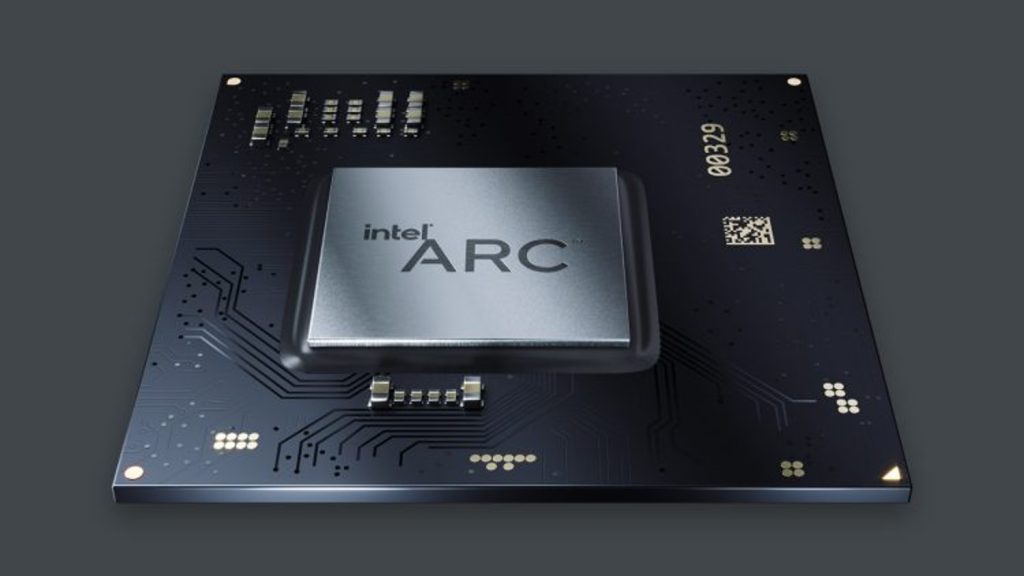This image depicts a detailed rendering of an Intel computer chip set against a solid all-black background, isolated from any surrounding components. The chip itself is predominantly black with a standout feature: a raised, metallic silver square positioned off-center. Embossed on this shiny silver core are the words "Intel" and "ARC," with "Intel" in small print at the top left and "ARC" in larger, all-capital letters below. Surrounding the silver square on the black processor are various gold electronic components and wiring paths, including a scannable feature and the numbers "00329" prominently displayed on the upper right side of the chip, likely indicative of a part number. The chip is seen from an angle, as if viewed from the lower left corner but in an aerial perspective, allowing a detailed view of the intricate circuitry and small transistors characteristic of such a processor.